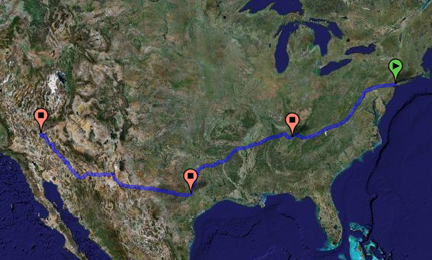This image depicts a detailed map of the United States of America, highlighting the country's geography with emphasis on greenery and topography rather than urban areas. The map appears to be a screenshot from a global mapping application, featuring a navigated path resembling a GPS route. This route is punctuated by several pinpoints: one in the western United States, one in the southern region around Texas, another in the midwestern area possibly near Kansas, and the final one in the eastern part, likely around New York or Boston. The path is color-coded—three red pinpoints mark the western, southern, and midwestern locations, while the easternmost pinpoint is green. The entire route is depicted with a connecting blue trail.